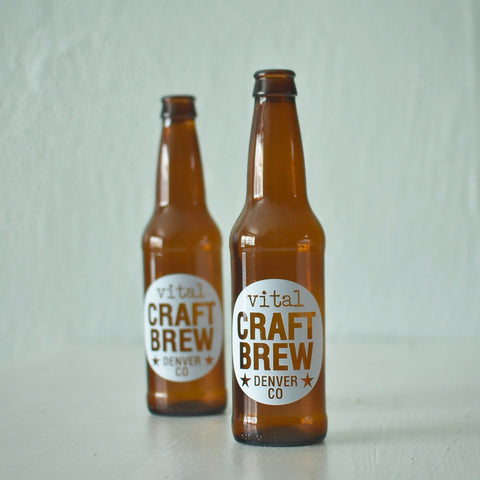This detailed color photograph depicts a pair of identical amber-colored, empty beer bottles displayed on a plain white surface against a subtly textured, off-white background. The bottles, which lack caps, prominently feature a white circular label positioned on their front. Within this label, the text "vital" is rendered in all lowercase letters, followed by "CRAFT BREW" in block uppercase letters. Beneath this, "DENVER, COLORADO" is printed in block capital letters, flanked by a five-pointed star on either side of the word "DENVER." The front bottle is more prominently displayed and in clearer focus, positioned slightly ahead and to the right of the other bottle, which appears more blurred and sits further back to the left. The overall setup highlights the modern design and branding of the beer bottles, emphasizing their transparent, amber-hued glass and the distinctive label detailing their origin from Denver, Colorado.